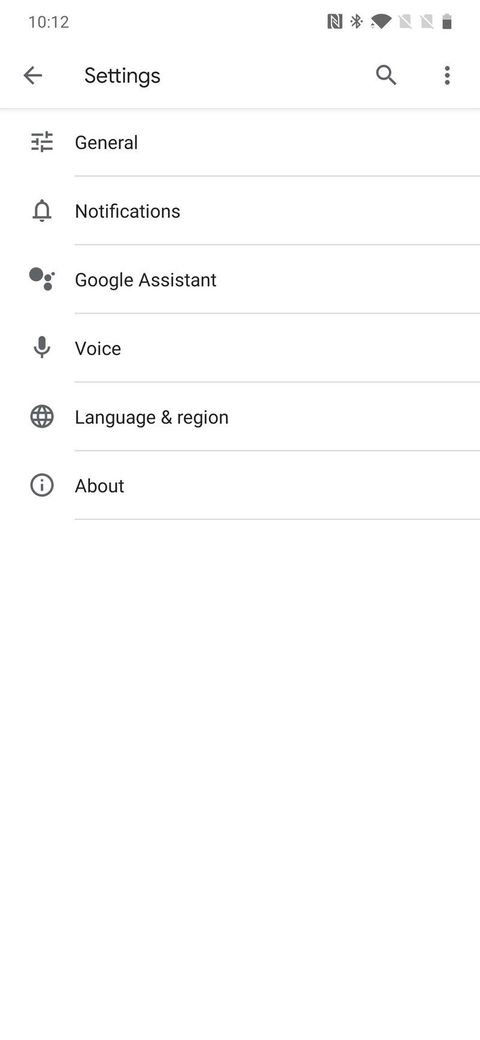In the top left corner of the image, the time is displayed as 10:12 in a light gray font. Moving to the center-right, there's an icon resembling an upside-down triangle or a handheld fan, also in gray. Directly below this icon, there's a small left-pointing arrow followed by the word "Settings", a magnifying glass, and three vertical dots. Each element is underscored by a line. On the next row, the label "General" appears with three horizontal lines beside it. Below this are "Notifications", accompanied by an image of a bell to the left. Continuing downward, "Google Assistant" is listed next, followed by "Voice", which is illustrated with a microphone icon. Further down, "Language and Region" is displayed next to a globe-like circle, featuring vertical and horizontal lines. This option is also underlined. Finally, at the bottom, the word "About" is shown, with a gray circle to its left containing a white, lowercase 'i' inside, outlined in gray.